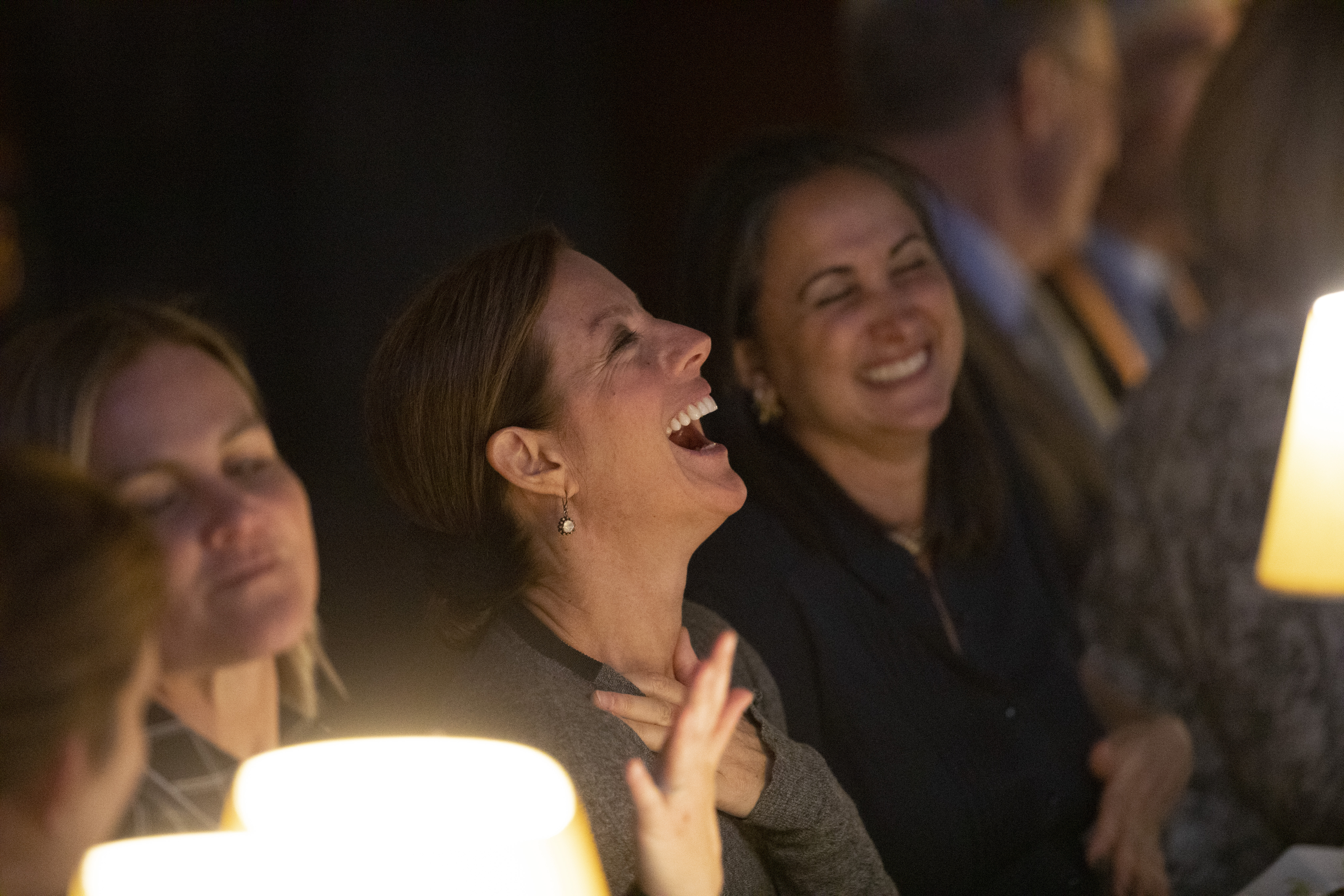The image captures a lively scene of a group of women seated in a row, deeply immersed in shared laughter. The central focus is on an older woman with brown hair tied back, wearing a dark gray sweater and dangly pearl earrings. Her joyous expression is vividly depicted as she clasps her hands to her chest, mouth wide open in laughter. Beside her, another woman dressed in navy blue has her hand on her stomach, displaying a broad smile. To the other side, a woman with a more subdued, closed-mouth smile is also caught in the moment. The background is predominantly dark, highlighting the bright lighting provided by three side table lamps with cream-colored shades that cast a warm illumination on the laughing women. Blurred figures of two men are noticeable in the background, adding to the depth of the scene, which appears to be set in a dimly lit, cozy environment possibly suggesting a comedy show or similar social gathering.